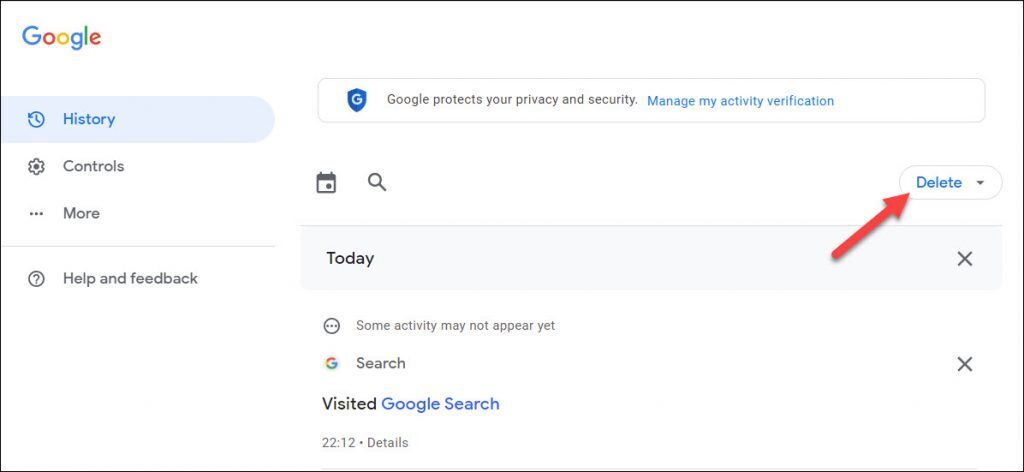Here is an example of a cleaned-up version of the caption you provided:

On a white background in the top left corner, there's the Google logo in rainbow colors. Below it, on the left side, the word "History" is highlighted. Next to it, there's a reverse arrow icon forming a counter-clockwise circle. Beneath that, there's a control widget and a "More" option represented by three dots, followed by a thin gray dividing line. Below the line, there's a question mark inside a circle with the label "Help and Feedback."

Centered on the screen is a "G" badge accompanied by the text "Google protects your privacy and security" in black, and a blue link reading "Manage my activity verification." This section is encapsulated by a box. Below this section, on the right, there is a calendar and a search bar. To the far right, there's a dropdown arrow shown in red labeled "Delete."

Underneath these elements, in bold, is the word "Today," which has an "X" icon to the right. Below that, a message reads: "Some activity may not appear yet," accompanied by an icon of three dots within a circle. Further down is a "G" icon next to a search input where users can exit.

Finally, beneath all this information, there's the word "Visited" in black text followed by "Google Search" in blue, and a timestamp—22:12—along with a "Details" link.

The only colored elements in this predominantly white interface are the Google logo, the red delete dropdown arrow, the Google search text, and the badge link.